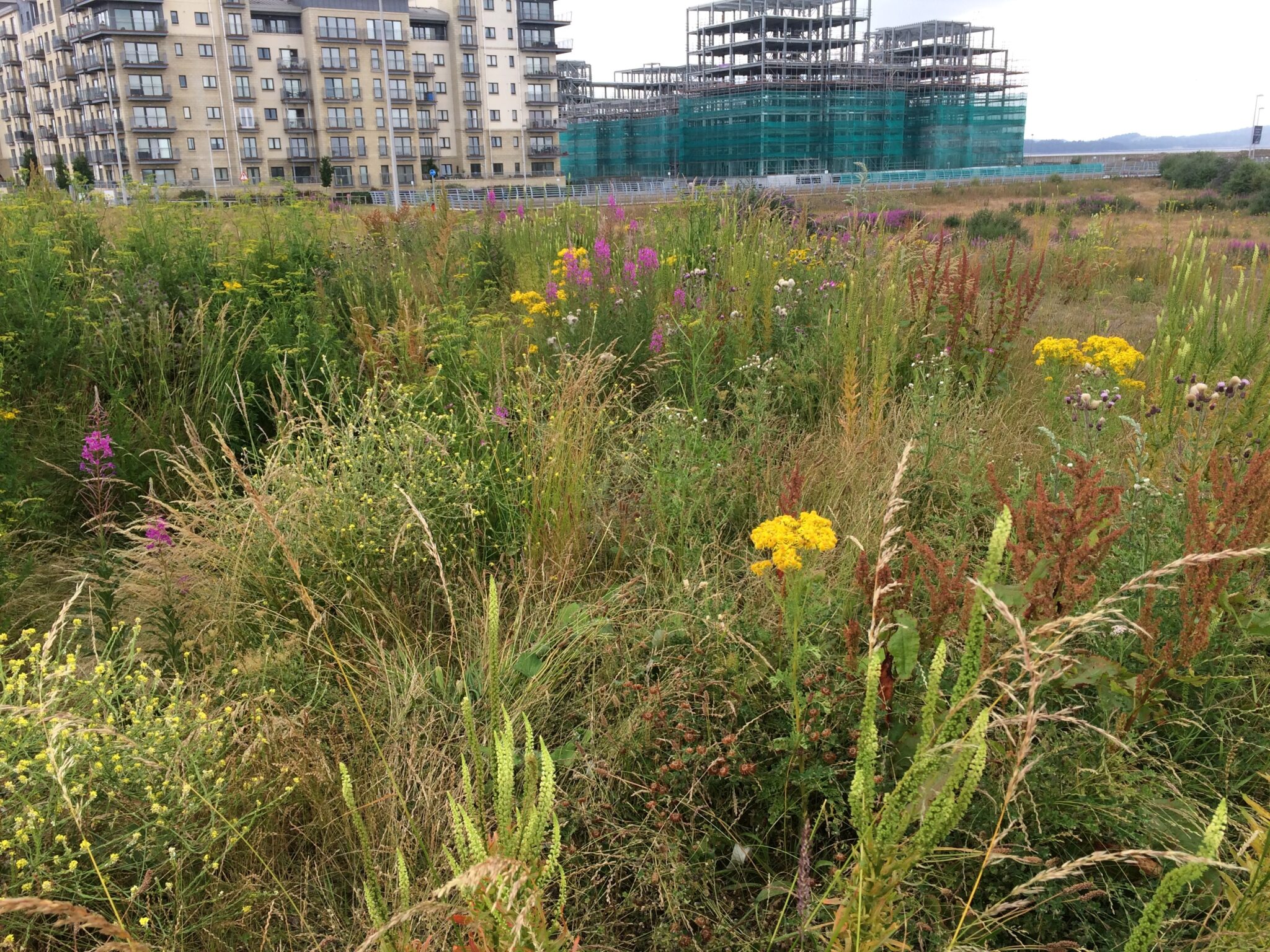This photograph captures an expansive, overgrown meadow filled with wildflowers and various plants. The lush field is awash with a vibrant palette of colors, including yellow and purple flowers, tall pink blooms, and brownish wheat-like plants, all surrounded by wild grasses and weeds. At the meadow's boundary in the distance, a metal fence demarcates the field from surrounding properties. Dominating the upper left corner of the image is a towering apartment complex with cream-colored exterior walls, abundant windows, and multiple balconies, spanning at least six to seven stories tall. Adjacent to it, situated slightly to the right and a bit closer to the foreground, is an active construction site with gray steel scaffolding and blue-green base structures, indicating the build of another apartment complex. In the far distance, a slight mountain ridge can be seen, adding a subtle yet striking backdrop to this richly detailed landscape.